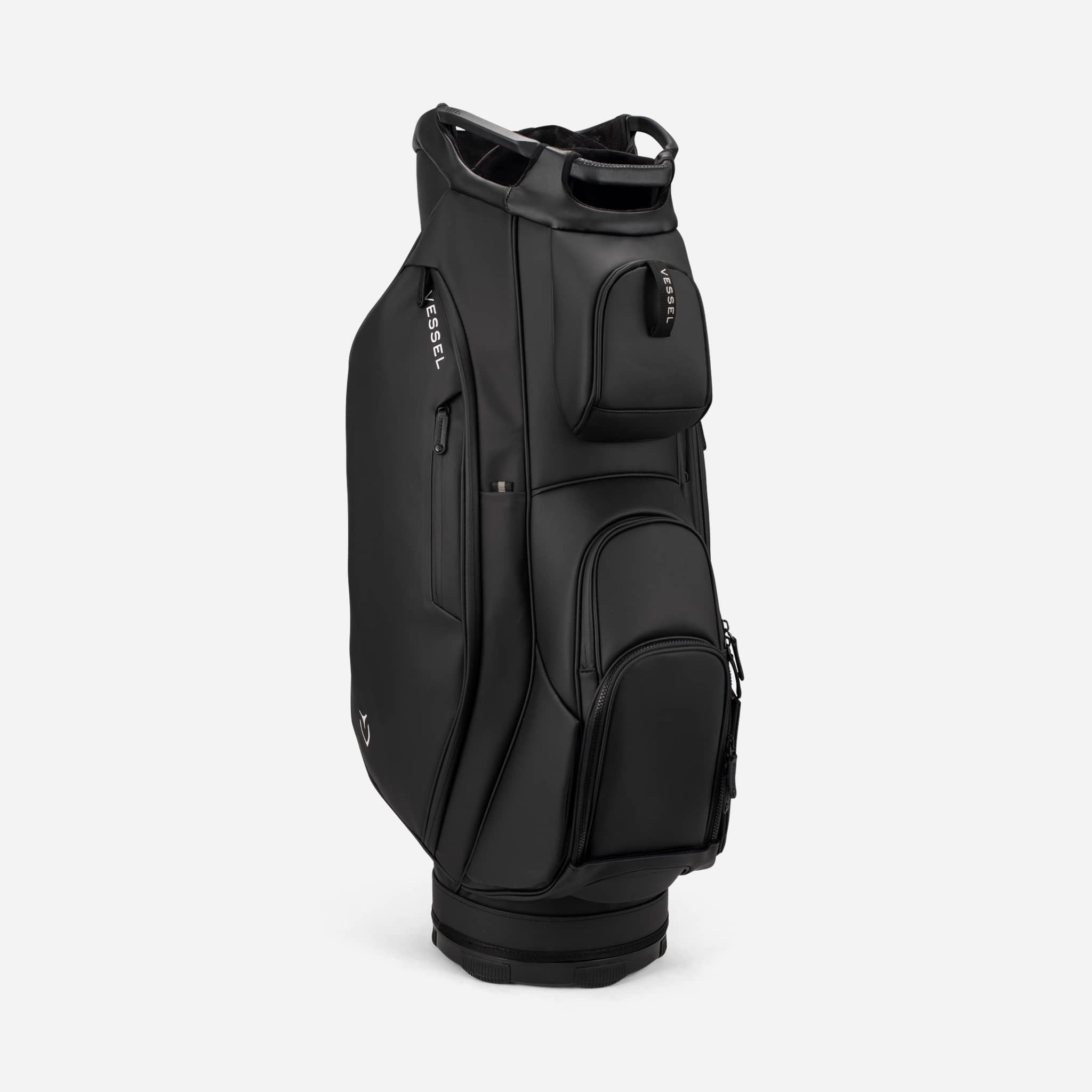On an off-white background, a sleek black golf bag is prominently displayed. The bag, devoid of golf clubs, features multiple zippered compartments, indicative of ample storage space. A label on the left zippered part near the bottom states "VESSEL" in white capital letters, while another tag hanging down from the back reiterates the brand name. The bag’s design includes several accesible zippered areas, with some compartments varying in size; the top compartment is smaller compared to the one below it. At the top and bottom of the bag, there are handle-like openings on three visible sides, providing ease of handling. A distinctive V logo in a circle, possibly representing the Vessel brand, is also noticeable. The entire presentation, likely a stock image for a product listing, emphasizes the golf bag's all-black, almost leather-like aesthetic, highlighted only by the white branding.